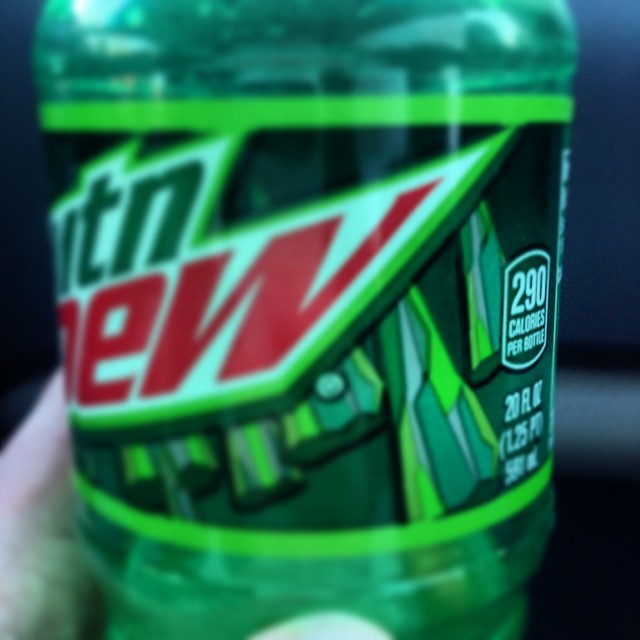The image depicts a Mountain Dew bottle with intricate details. At the top of the label, the word "Green" is prominently displayed, followed by "Dew" in red at the bottom of the label. The bottle itself exhibits a clear finish at both the top and bottom. Dominating the center of the bottle is a dark green label that features lighter green rectangles, adding a vibrant design element.

Additionally, there seems to be a pattern of triangular shapes on the label, reminiscent of stones. Nutritional information indicates that the beverage contains 290 calories per bottle. The bottle's capacity is specified as 20 fluid ounces, which is equivalent to approximately 1.25 liters. The surface of the bottle appears to be reflective, enhancing its visual appeal.